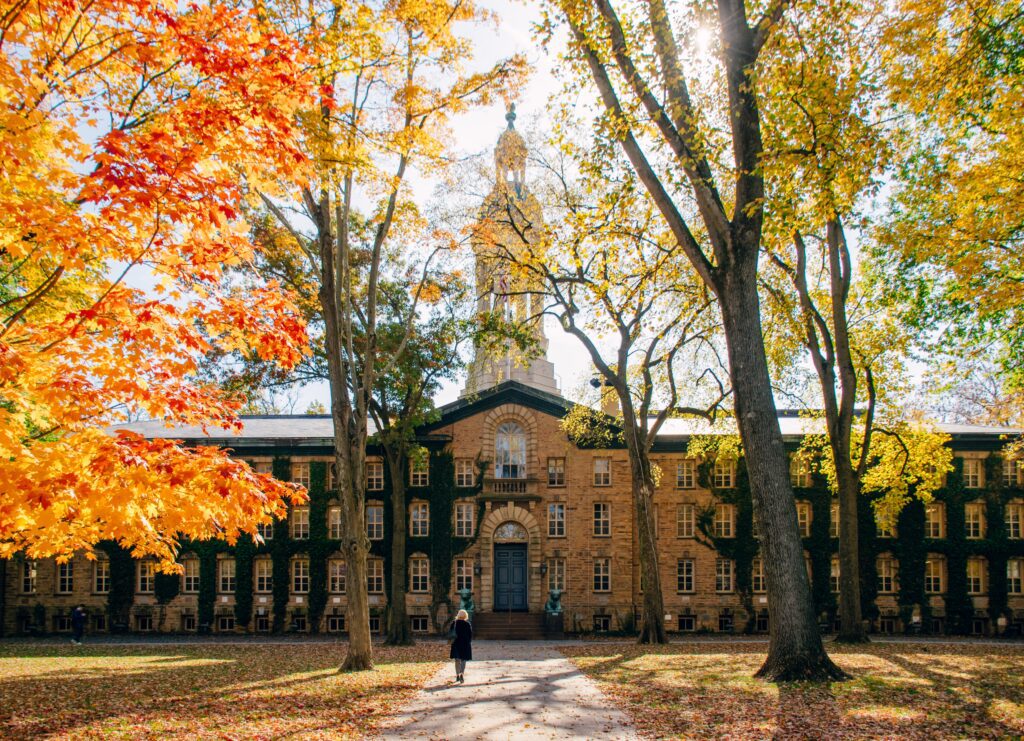In this image, an official-looking brick building, possibly part of a college or university, stands prominently against an overcast sky. Its architecture is accentuated by a brown brick archway framing a blue door, above which is a window or balcony. Extending from the building's center is a white bell tower that reaches towards the sky, hinting at the structure's institutional significance.

The façade of the building is adorned with meticulously trimmed ivy or vines, forming a crosshatch pattern around the numerous windows. In front of the building, a wide sidewalk bordered by lush grass and scattered leaves leads directly to the entrance. The autumn season is unmistakable, with the tall trees flanking the pathway displaying a vibrant palette of green, yellow, orange, and red leaves. Many of these leaves have fallen, creating a colorful carpet on the grass.

A woman in a black jacket, with blonde hair, is seen walking towards the building, adding a human element to the scene. The entire setting is bathed in the muted light of a cloudy day, with the sun subtly illuminating the grass and enhancing the autumnal colors. Additionally, the large building has a sense of continuity, either through an adjoining structure or as part of a larger complex, emphasizing its grandeur and university-like ambiance. This picturesque, timeless scene evokes the charm and tranquility of an academic institution in fall.